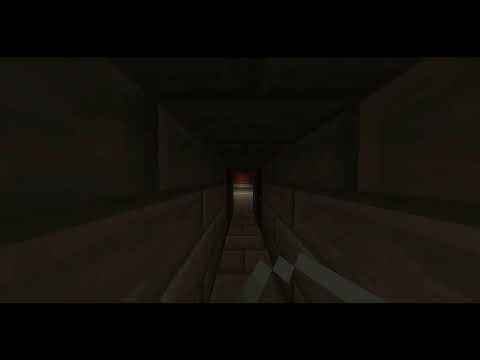The image is a darkened screenshot from a video game that resembles Minecraft, characterized by its low-resolution, polygonal graphics. The scene features a narrow, low corridor lined with large, dark gray and shaded, dull red or rusty red bricks, creating the walls, floor, and ceiling. The player's first-person view shows them holding a tool, likely a pickaxe or bladed weapon, positioned close to the center vertical line and slightly to the right. The corridor, which occupies most of the dimly lit image, leads to a faintly illuminated area suggesting a room with a light source casting dim light onto the floor and a red wall visible in the distance. The overall darkness and absence of light sources make it challenging to discern the finer details of the scene.